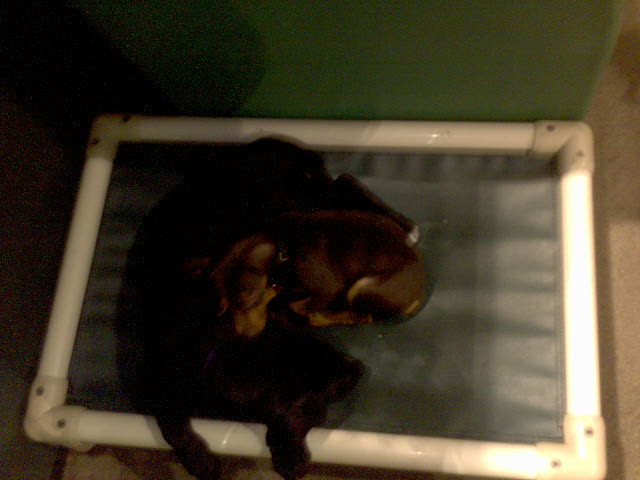The image portrays a pair of Dobson bloodhounds, one larger and one smaller, nestled together in a unique, rectangle-shaped dog bed constructed from PVC pipes and elbows. Due to the poor lighting and the dark color of the dogs' fur, their precise details are challenging to discern. The larger dog lies on the bed's tarp-like bedding material, which has a grayish hue, while the smaller puppy, dark brown in color, rests atop the larger dog, with its two front paws extending over the front edge of the PVC frame. The scene is set against a green wall with manila-white carpeting beneath the bed. Despite the blurry and dark conditions, a sliver of natural light from the right casts faint shadows, adding a slight definition to the forms of the dogs and the bed.